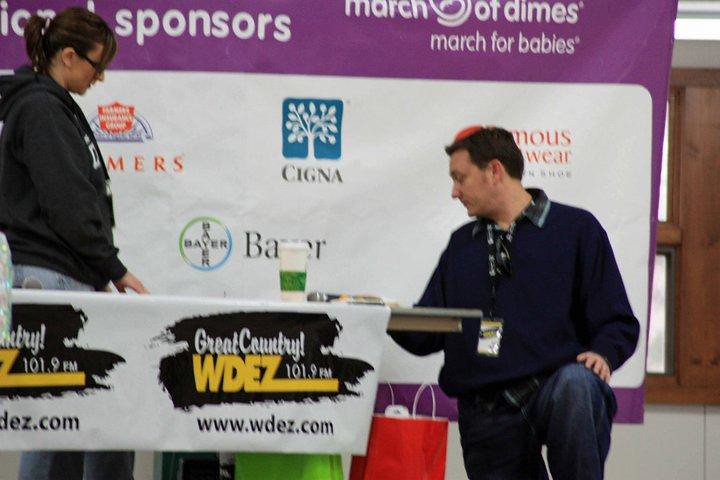In this detailed photograph, two people are positioned in front of a purple banner adorned with various sponsor logos, indicating a charity event, possibly the March of Dimes March for Babies. On the right, a Caucasian man, wearing a blue windbreaker over a green and blue plaid shirt and blue jeans, is crouching down with a badge around his neck and his hand resting on his thigh. To the left, a Caucasian woman in a blue hoodie, gray sweatpants, and glasses with her dark hair tied back in a ponytail, stands behind a table. Both are gazing at a white coffee cup with a green stripe, which is on the table. The table bears a banner that reads "Great Country WDEZ 101.9 FM" with the website "www.wdez.com" underneath. Below the table, two gift bags, one red and one green, can be seen. The backdrop features a central white square with notable sponsor logos, including a white tree on a blue background for Cigna, alongside emblems from Farmers Insurance, Famous Footwear, and more. A partially obscured red logo is also noticeable behind the man's head.